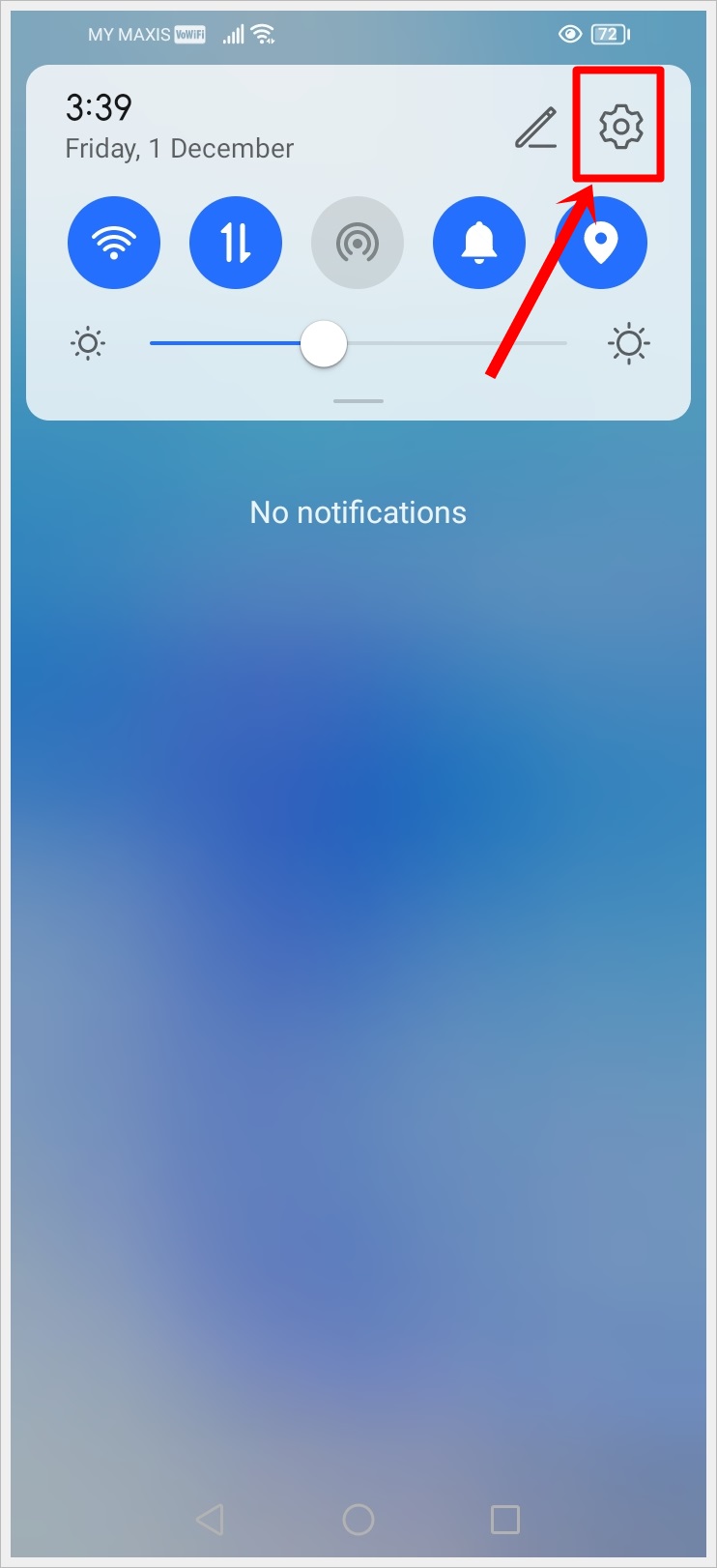The image appears to be a screenshot taken from a cell phone, set against a predominantly blue background that varies in shade: darker blue in the center, lighter bluish-gray in the lower-left corner, and a medium blue elsewhere. At the top of the screenshot, the text "My Maxis" is displayed, with the time "3:39" indicated in black font. It also shows "Friday" and the date "December 1." To the right of the time, there's a nearly full battery icon. An image of a settings wheel icon, outlined in a red square, is located towards the right side. An arrow extends from this red square, pointing to it from the top left, indicating focus on the settings wheel. Below, a blue circle with lines denotes the volume control, next to another blue circle featuring a bell icon, which suggests notifications. There is also a brightness adjustment bar, positioned slightly to the left of the center, indicating average screen brightness. Underneath these elements, white text states, "No Notifications," signifying that there are no active notifications on the device.